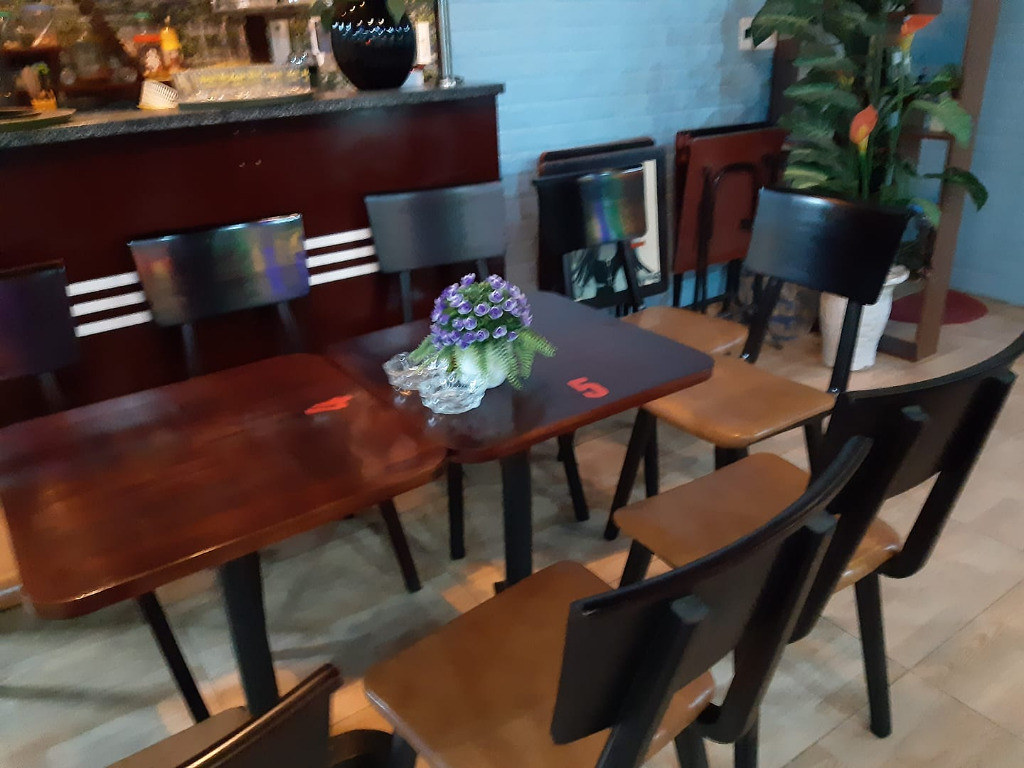This is a slightly blurred photograph of a modernistic, minimalist dining setup, likely within a restaurant or cafe. The scene features two glossy mahogany brown tables pushed together diagonally from bottom left to top right, adorned with numbers 4 and 5 in orange or red. The number 5 table holds a potted bouquet of purple flowers with green leaves, placed in a white bucket along with two glass ashtrays. Surrounding the tables are six to eight chairs, each with dark beige seats, black wooden backs, and black legs. The room has a cream-colored tile floor patterned with large squares, and behind the table setup, in the upper left, there is a buffet cabinet with a gray countertop cluttered with blurred vases, urns, and platters. The cabinet, dark mahogany with white bars across the bottom, further adds to the modern decor. The background features a blue wall, and in the upper right, there's a large white vase on the floor next to a tropical rubber plant with orange blooms. Nearby, a stack of folded TV trays rests against the wall. The countertop visible in the background suggests a bar area, characterized by three white stripes running across its front and some glassware and a black vase on top.